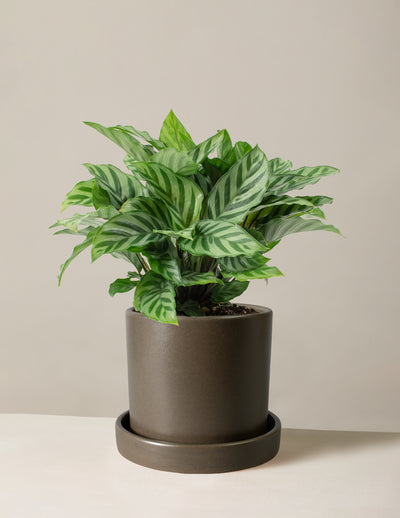In the image, there's a healthy-looking potted plant, sitting on a white surface against a light beige or gray wall. The pot is dark brown, resembling coffee, and rests on a matching circular base that appears to catch water. The plant itself is bushy with numerous large leaves that are light green with distinctive dark green stripes or veins, giving them an almost tiger-striped appearance. The leaves are oval-shaped and point in various directions, creating a full, compact look. The pot displays brown soil, adding to the natural and robust appearance of the plant. The overall composition suggests either a very well-maintained live plant or a high-quality artificial one due to its vibrant and healthy form.